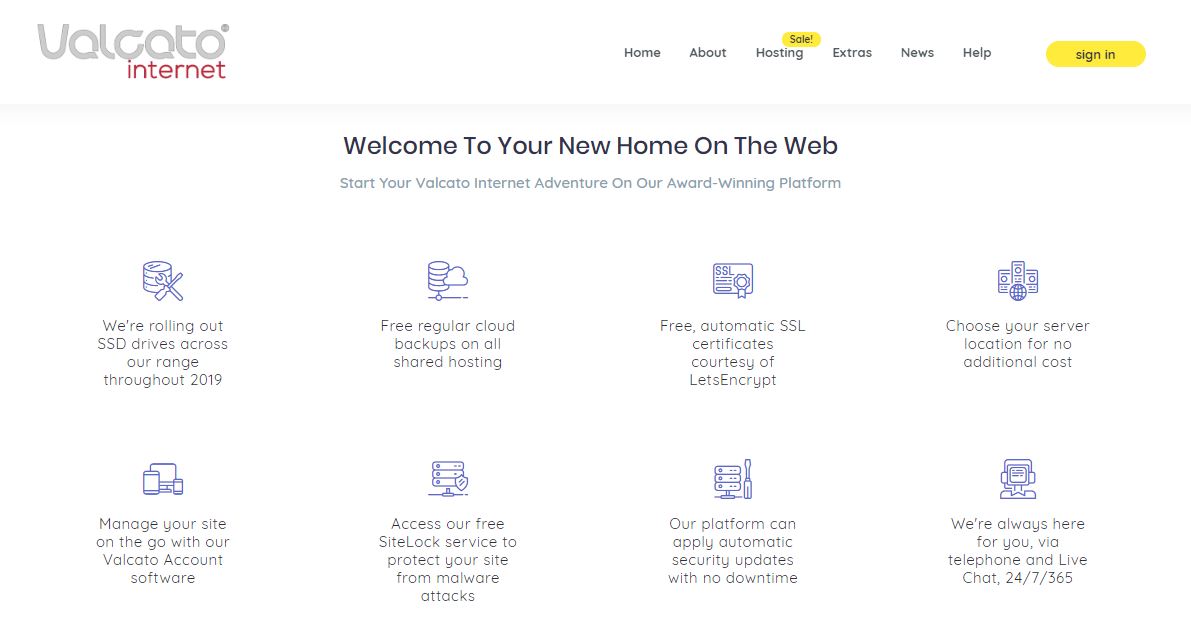Welcome to Your New Home on the Web

Experience the future of browsing with Val Kato, presented in a sleek, easy-going grey font designed for a smooth and stylish user interface. The top navigation menu includes essential links such as Home, About, Hosting, Extras, News, and Help, accompanied by a user-friendly sign-in section.

Welcome to your Val Kato Internet adventure, where our award-winning system offers a plethora of features to enhance your online experience:

- **Home, About, Hosting, Extras, News, Help:** Navigate easily through our comprehensive menu at the top.
- **Rolling Out SSD Drives:** Enjoy faster performance with our extended range of SSD drives.
- **Free Regular Cloud Backups:** Safeguard your data with automatic cloud backups at no additional cost.
- **Free Automatic SSL Certificates:** Secure your site with SSL certificates provided by Let's Encrypt.
- **Choose Your Server Focus:** Customize server settings according to your specific needs without extra charges.
- **Manage on the Go:** Control your site anywhere, anytime with our Val Kato account software.
- **Free Site Lock Service:** Enhance your site's security with our complimentary Site Lock feature.
- **Automatic Security Updates:** Implement security updates seamlessly with no downtime to ensure your platform stays protected.

We're committed to providing exceptional support, reachable via phone or chat for any assistance you need. Your journey with Val Kato promises to be secure, efficient, and always at your fingertips.